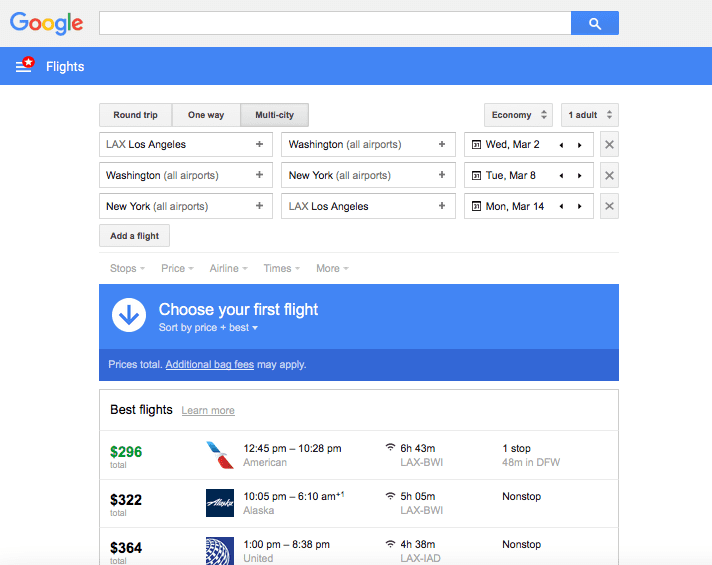The interface showcases a search tool for booking flights. At the very top, there is a light gray rectangle featuring Google's multicolored logo on the left. Adjacent to this logo is a white input field bordered by a slightly darker gray, intended for search entries. Beside this field is a blue rectangle with a magnifying glass icon. Below, there is a long blue rectangle with three horizontal lines. Partially covering the top line is a red circle with a star, labeled "Flights."

Underneath are several interactive options displayed as gray rectangles outlined in darker gray. The options include "Round Trip," "One Way," and "Multi-City." To the right, there are two more interactive fields: one that reads "Economy" with up and down arrows, and another that says "One Adult" with similar arrows.

Below this are flight detail fields. The first white rectangle (outlined in black) indicates "LAX Los Angeles" with a plus sign. Another field reads "Washington All Airports," also accompanied by a plus sign. A calendar icon displays "WED, MAR 2," flanked by navigation arrows. A light gray rectangle with an 'X' symbol appears on the side.

Further details follow:
1. The left-hand side shows "Washington All Airports" with a plus sign, "New York All Airports" with a plus sign, a calendar saying "TUE, MAR 8," navigational arrows, and another 'X' in gray.
2. A similar layout features "New York All Airports" paired with a plus sign, "LAX Los Angeles" with another plus, and a calendar showing "MON, MAR 14" with additional arrows and 'X.'

There's an additional gray rectangle labeled "Add a Flight," followed by sorting options: "Stops," "Price," "Airline," "Times," and "More," each with downward-pointing arrows. A blue rectangle encourages users to "Choose Your First Flight," sorted by "Price" and "Best," accompanied by another arrow.

Information regarding total prices appears in a darker blue rectangle stating "Prices Total, Additional Bag Fees May Apply." Below, a black-outlined rectangle details "Best Flights" with a "Learn More" link. Each flight option is summarized:

1. Priced at $296, a flight featuring an eagle logo (red and black wings), departing at 12:45 PM and arriving at 10:28 PM on American Airlines, includes Wi-Fi, and spans 6H 43M from LAX to BWI with a 48-minute stop in DFW.
2. Another at $322 on Alaska Airlines, priced in a blue rectangle, departs at 10:05 PM and arrives at 6:10 AM with Wi-Fi, and is a 5H 05M non-stop flight from LAX to BWI.
3. Priced at $364, a United Airlines flight with a logo depicting a planet, departs at 1:00 PM and arrives at 8:38 PM, includes Wi-Fi, and spans 4H 38M non-stop from LAX to IAD.

Overall, the interface detailed provides a comprehensive layout for selecting and reviewing flight options efficiently.